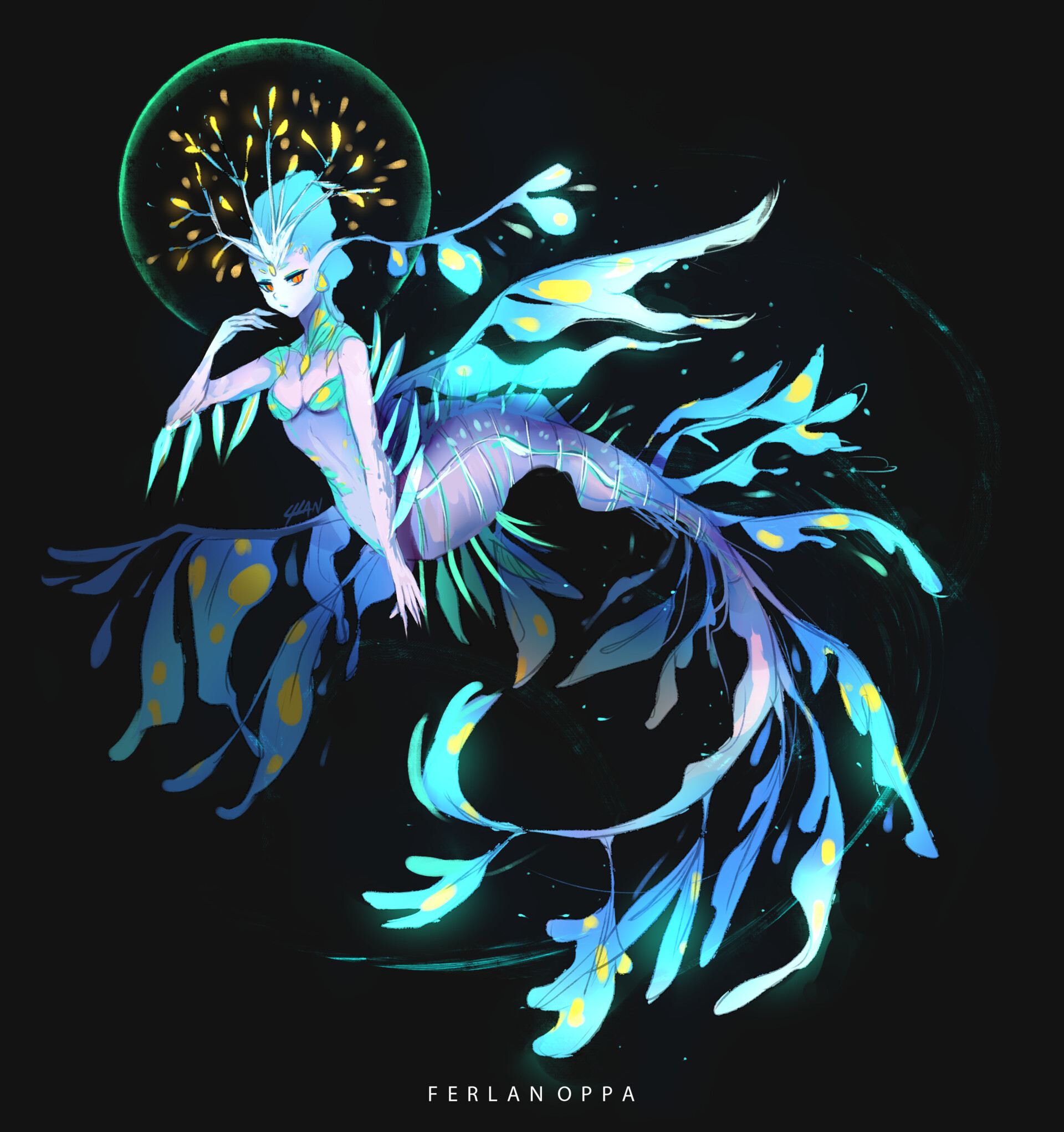This striking digital illustration showcases a female figure in an imaginative blend of fairy and mermaid characteristics against a solid black background. Her upper body appears fairy-like, with light purple skin, almost white face, and elaborate teal blue hair piled on top of her head. Unique to her look are the branches growing from her forehead, adorned with yellow leaves, and encircled by a green halo. Her wings and ear take the form of long, delicate fins.

The synergy of her form transitions into a mermaid's tail, primarily dark purple, which gradually morphs into an array of patterned frills and fins in vivid colors like mint, white, light blue, dark blue, purple, and yellow. This tail is detailed with yellow polka dots, enhancing its fantastical appearance. She holds one hand elegantly just below her mouth while the other hangs straight down. The lower body features elements resembling leaves, amplifying the mythical essence. 

The illustration includes the name "Ferlanoopa" in bold white letters at the bottom, hinting at an intriguing character whose details beckon further exploration.